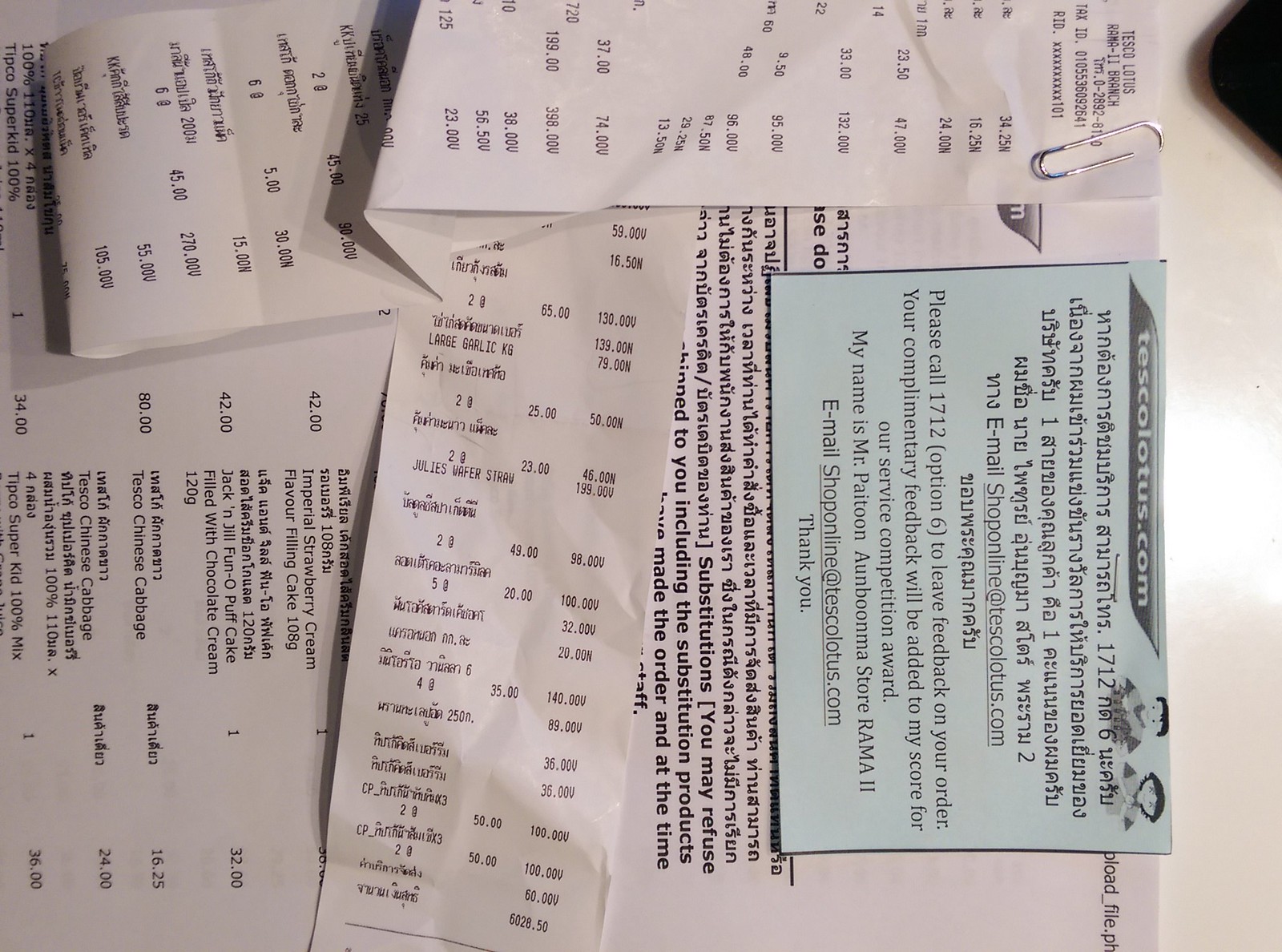The photograph is a close-up of a collection of various receipts and papers that are either paper-clipped or stapled to the top of a white piece of paper with extensive black text in both Arabic and English. A prominent blue rectangle paper is also stapled, which includes a message requesting feedback on a grocery order, specifying, "Please call 1-712-OPTION-6 to leave feedback on your order. Your complimentary feedback will be added to my score for our service competition award. My name is Mr. Paitoon, Store Rama 2." The email provided is shoponline@tescolotus.com, and it ends with a thank you note. Among the receipts listed in both languages, various grocery items such as large garlic, Chinese cabbage, Jules Wafer Straw, puff cake filled with chocolate cream, and various other products can be identified. The receipts provide detailed information about the items purchased, including quantities and prices, highlighting an array of groceries bought from the store.